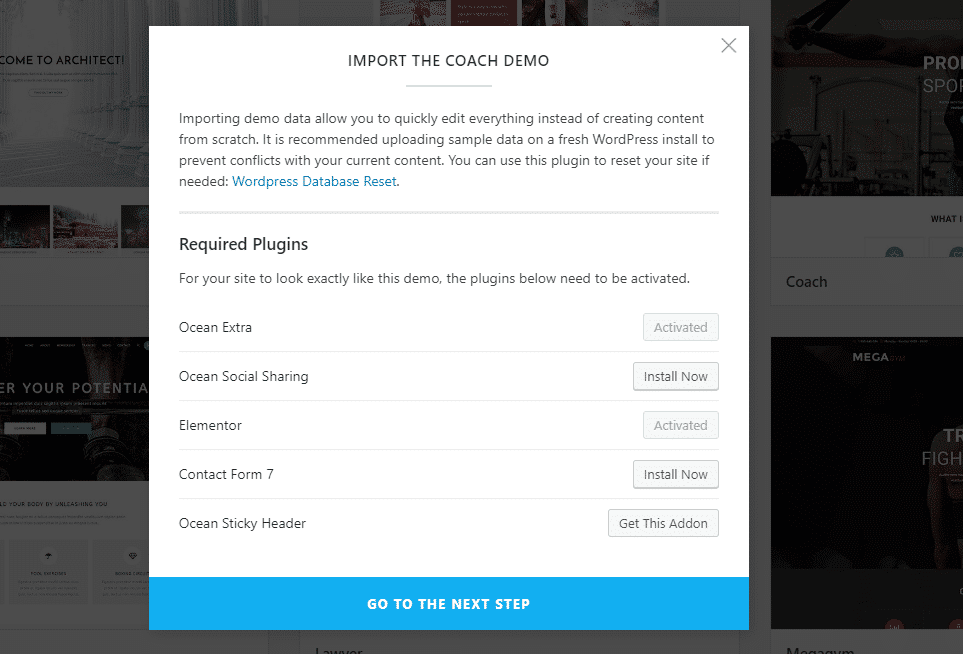In the background, the image displays several sections illustrating the process of importing the Coach Demo. Importing demo data is highlighted as an efficient way to quickly edit various elements without having to create content from scratch. The recommendation to upload sample data on a fresh WordPress install is emphasized to avoid conflicts with existing content. 

A suggestion to use a plug-in called "WordPress Database Reset," which is color-coded in blue, is given for those who may need to reset their site. 

Highlighted below are the required plug-ins needed for the site to look exactly like the demo:
- "Ocean Extra" is shown as activated.
- "Ocean Social Sharing" with an "Install Now" button.
- "Elementor" is also marked as activated.
- "Contact Form 7" with an "Install Now" button.
- "Ocean Stickers Header" has a prompt to get this add-on.

In the lower portion of the image, there is a blue rectangle with white text that reads, "Go to the next step."